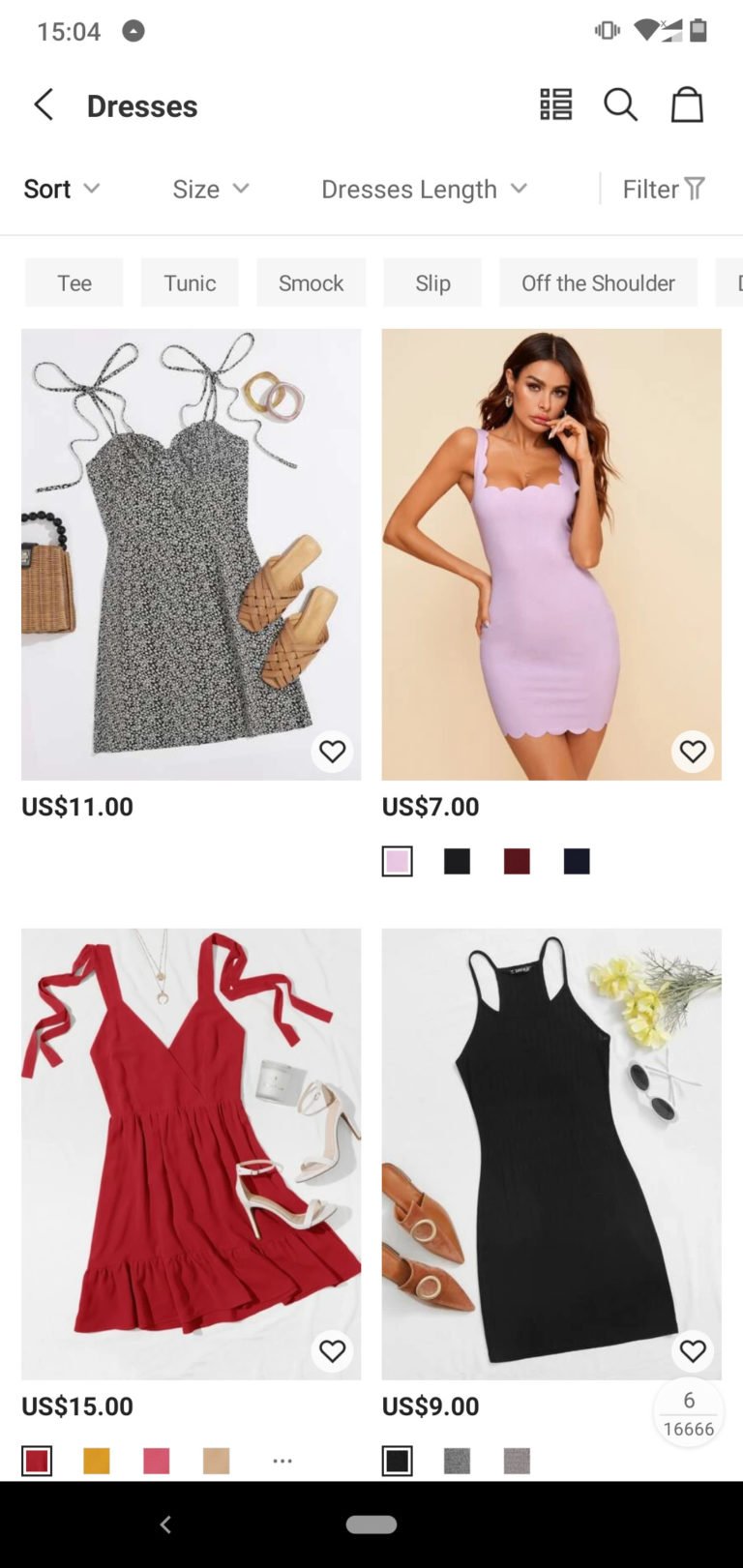The screenshot displays a fashion e-commerce website specializing in dresses. At the top of the screen, the time reads "15:04" with indicators for Wi-Fi (currently unconnected with an 'X' through it) and battery life. Below the time, there is a left-pointing arrow and bold text that reads "Dresses." Adjacent to this, there are icons including a series of squares and rectangles, a magnifying glass, and a picture of a purse. 

Underneath the title "Dresses," two bolded options, "Sort" and "Size," are accompanied by drop-down boxes, although the "Size" option is currently grayed out. Another drop-down menu titled "Dresses length" allows users to choose the desired length of the dresses. Additionally, a "Filter" button is present for further customization.

Beneath these options, from left to right, there are buttons labeled "T," "Tunic," and "Smock." Below these, four different dress options are showcased:

1. The top-left dress is a taupe-colored, skinny-strap dress with a checkered pattern, priced in US dollars. It is shown both being worn by somebody and lying on the ground beside sandals.
2. A tight lavender dress worn by a woman, priced at $7.
3. The bottom-left dress features red straps and is priced at $15, with additional color options available in orange, brown, and black.
4. Lastly, a black dress priced at $9 is shown.